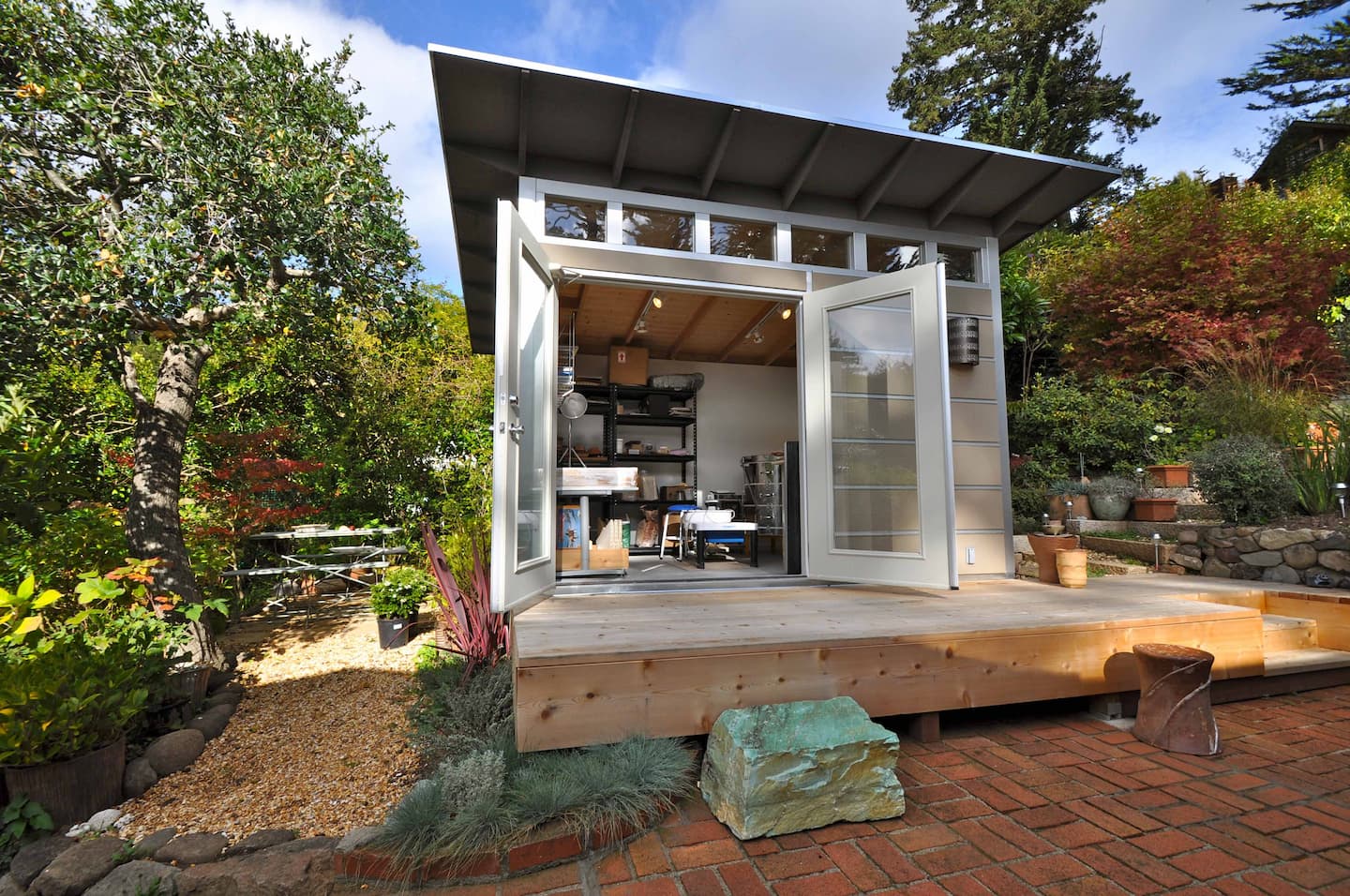The image features a small, well-constructed wooden platform surrounded by a beautifully maintained area with various trees, both green and red, under a clear blue sky with white clouds. The platform supports a square structure that could be a shed, tiny house, or even a music studio. The light brown wooden platform includes a porch and steps leading up to the building. The building itself is framed in gray with a distinct roof that overhangs on all sides. It has two doors, each with a single large window pane, and five rectangular windows above the doors. The windows are notably clean, enhancing the structure's meticulous and artistic design. Below the platform, there is a large square rock with a greenish hue on top, sitting on a surface made of red bricks with mortar in between. Adjacent to this rock is a rusted can. The left ground area sports light orange gravel and a couple of black potted plants, while the right side has several orange pots, some with white flowering plants. The interior of the building, visible through the open door, shows a cluttered room with a black metal shelf, objects, and possibly a fan or light attached to a wooden ceiling.